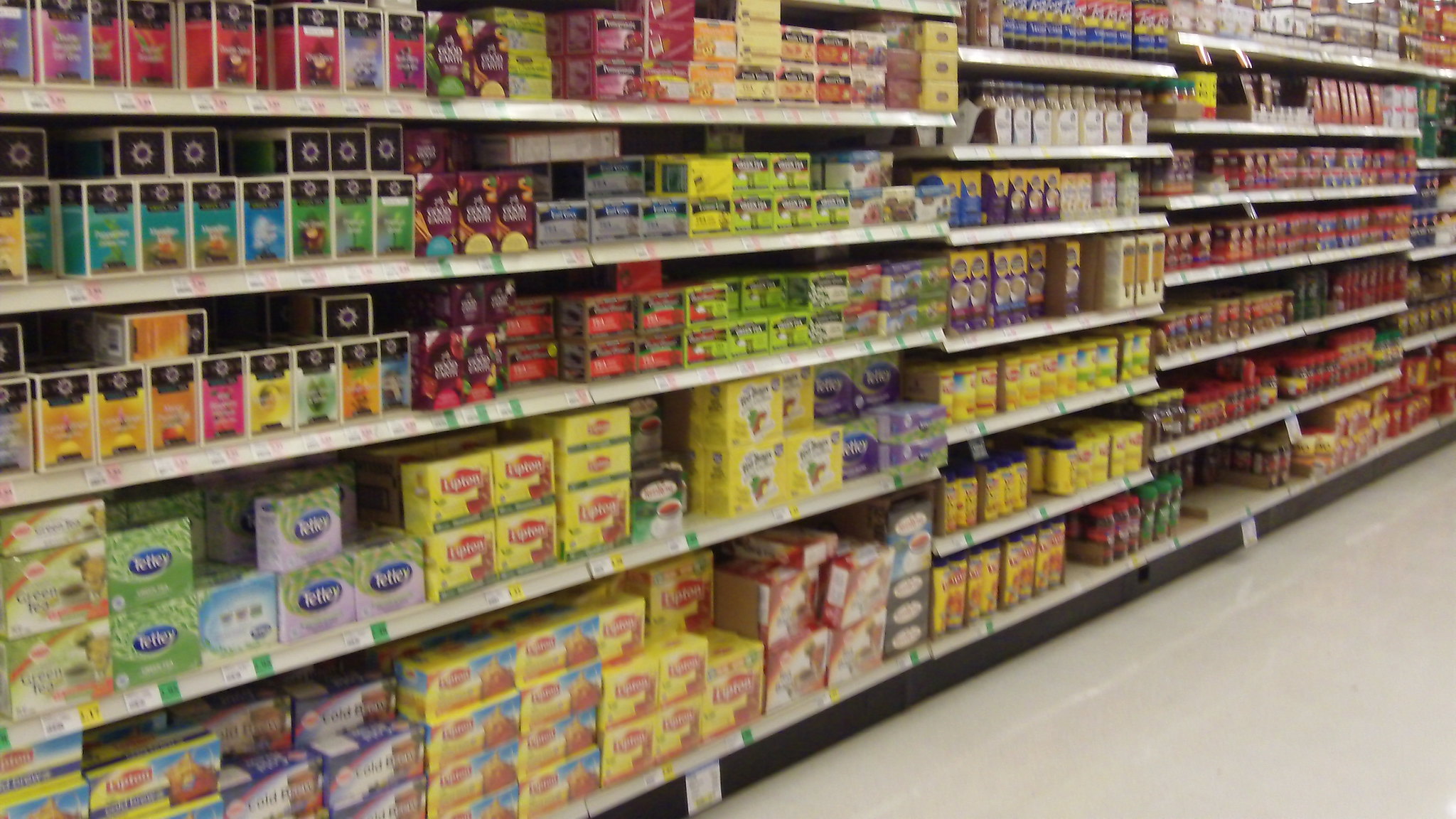The photograph depicts an aisle inside a grocery store, characterized by its standard overhead lighting, with no evidence of flash usage. The image, though slightly blurry, showcases a well-stocked shelf segment predominantly featuring a myriad of tea brands. On the left-hand side, prominently, Tetley and Lipton tea boxes are visible amongst a diverse collection of tea products including various green, black, and citrus-flavored teas. The tea boxes display a vibrant array of colors indicating the rich variety available. Moving towards the center of the image, the shelves continue with more products whose details are indistinguishable due to the suboptimal photo quality and angled viewpoint. Price tags hang above the items, although the numbers are unreadable. Overall, the scene captures the extensive and organized assortment typical of a grocery store tea aisle.